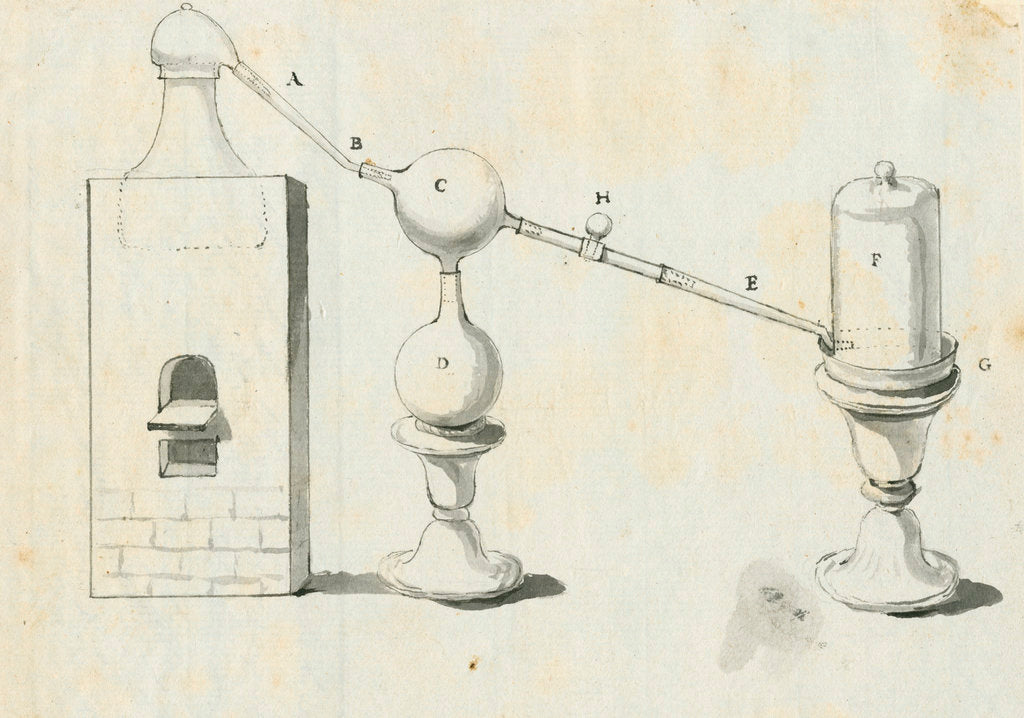This monochromatic ink illustration, executed with a brush on landscape-oriented, splotchy, white, and yellowed paper, depicts an intricate schematic with labeled components. On the left stands a tall, rectangular brick column with an arched opening, resembling a small pizza oven. At the top of this column, a pawn-shaped component, small at the top and wider at the base, is labeled A. A pipe descends diagonally from this element, labeled B, leading to a spherical flask labeled C, which is perched on another round flask labeled D, both resting on a candelabra-shaped stand. Another pipe, labeled H and E, extends diagonally down from flask C to a tall, cylindrical bell jar labeled F, situated on an ornate, chalice-like base labeled G. The entire image is characterized by hand-lettered labels and detailed ink shading, capturing the functional design of what appears to be a distillation apparatus.